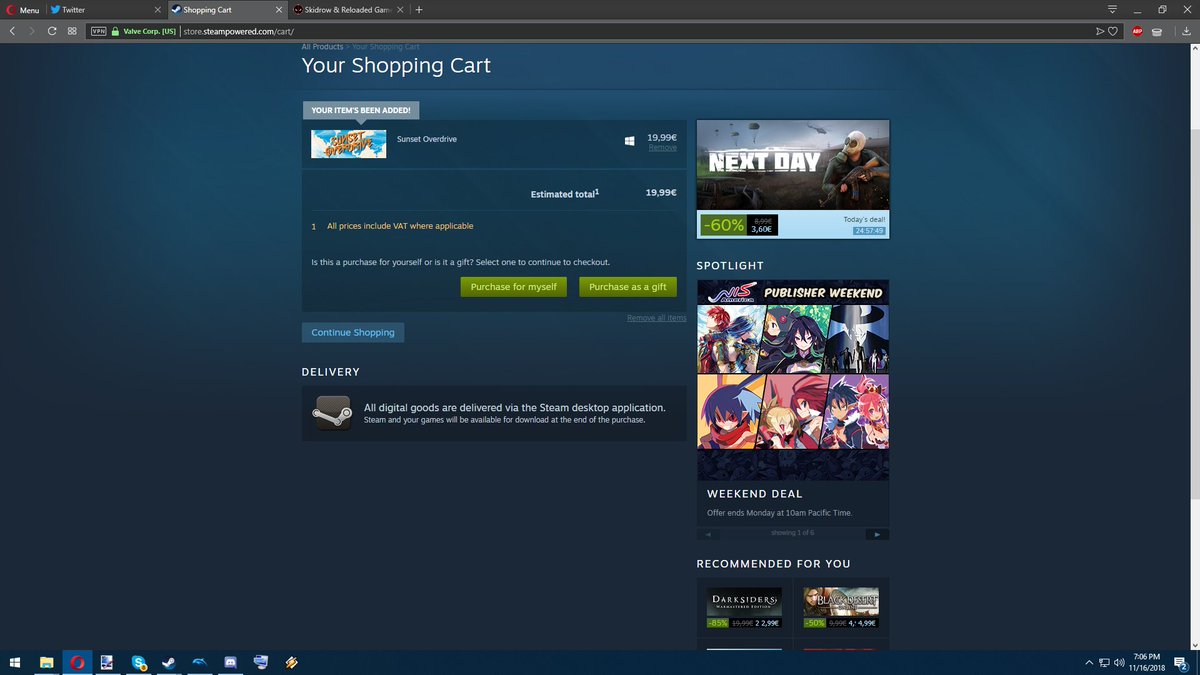The image showcases a computer screen displaying a shopping cart from store.streampower.com. The interface features a blue background with the prominent heading "Your Shopping Cart." It appears the user is on the tab labeled "All Products - Your Shopping Cart," implying they’ve recently clicked to view their cart.

Central to the screen is a confirmation message stating "Your items have been added," accompanied by a picture of the game "Sunset Overdrive," priced at $19.99. The estimated total also shows as $19.99. A notable detail is the yellow text clarifying, "All prices include VAT where applicable."

Beneath this, a white text prompt asks, "Is this a purchase for yourself or is it a gift? Select one to continue to checkout." There are two green buttons following this query: one labeled "Purchase for Myself" and the other "Purchase as a Gift." 

Below these options, there's a "Continue Shopping" button. Further down, a box marked "Delivery" explains, "All digital goods are delivered via the Stream desktop application. Stream and your games will be available for download at the end of the purchase."

On the right-hand side of the screen, there's a sidebar featuring various other games, categorized under "Spotlight" and "Recommended for You."